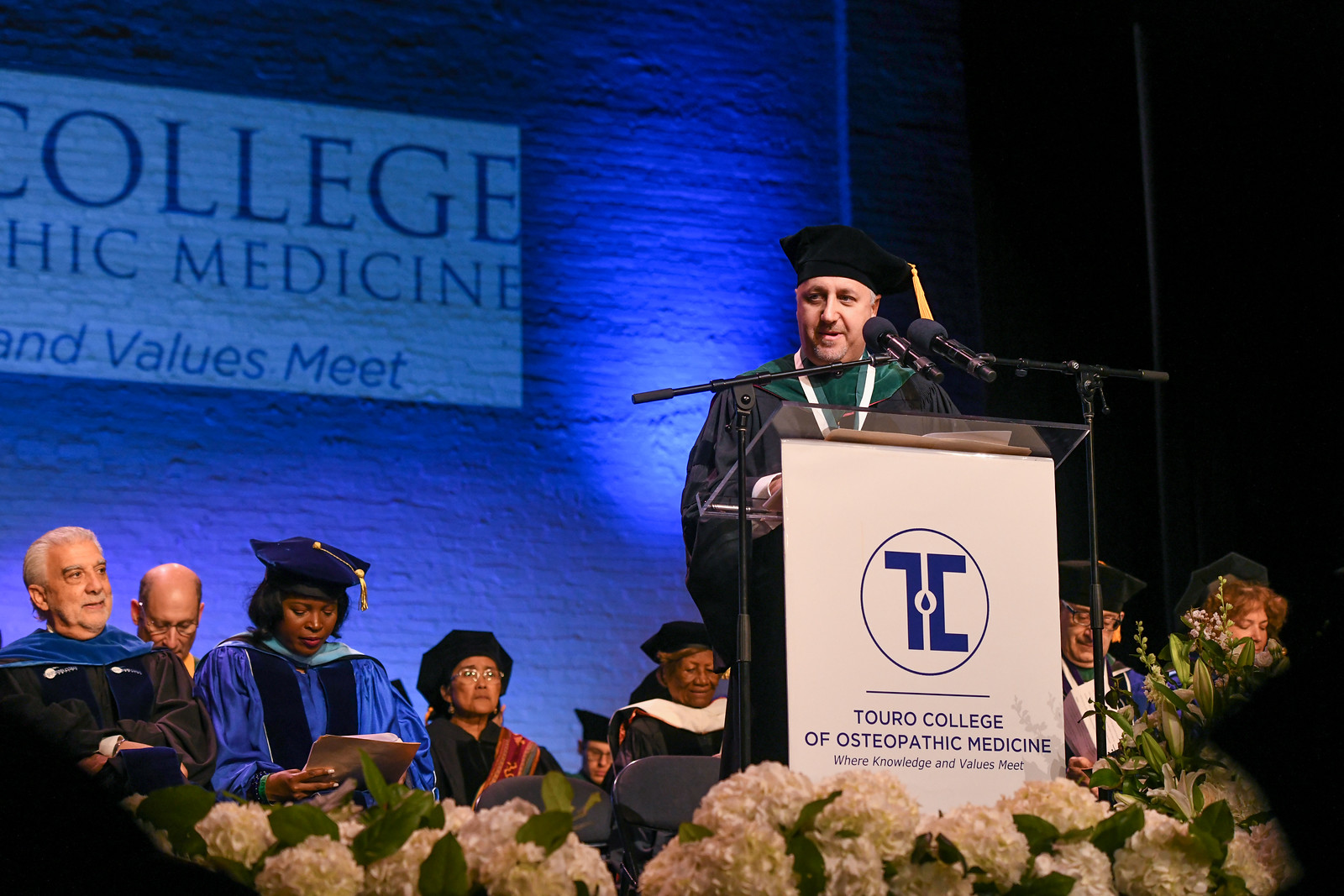In this color photograph, a graduation ceremony is taking place at Touro College of Osteopathic Medicine. The focal point is a speaker, presumably a professor, standing behind a clear glass podium adorned with a white sign. The sign features a blue logo encircled in blue and reads, "Touro College of Osteopathic Medicine, where knowledge and values meet." The professor is dressed in a traditional graduation outfit: a black gown with a green collar, a black mortarboard with a yellow tassel hanging on the left side, and is speaking into two microphones.

The backdrop of the scene includes a blue brick wall on the left, partially obscured by a projection displaying the text "College of HIC Medicine and Values Meet," although some parts have been cut off. On the right side of the stage is a black curtain. Seated behind the speaker are eight individuals who also appear to be professors or faculty members; some are wearing mortarboards, while others are not. Their gowns vary in color, with the women in blue gowns and the men in black.

In the foreground, a row of flowers decorates the bottom and right corner of the image, adding a touch of elegance to the ceremonial setting.